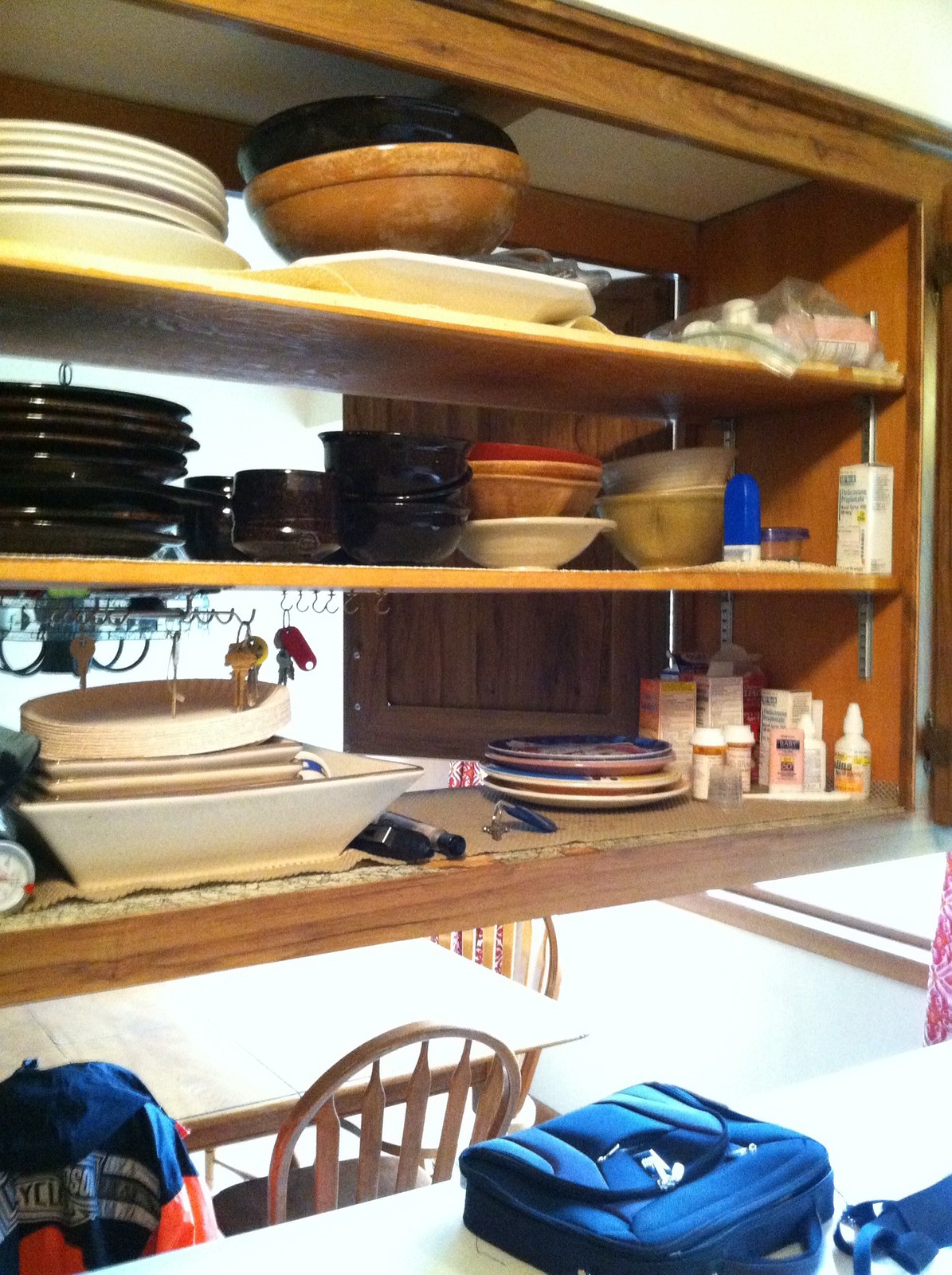The focal point of the image is a three-tiered wooden shelf, crafted from medium brown wood with distinct grain patterns. This shelf is mounted above a pristine white kitchen countertop. Resting on the countertop is a closed, black computer bag.

Starting from the top shelf, on the left side, there is a neatly stacked collection of white plates. Adjacent to these is a varied stack of bowls in alternating colors: black, brown, and white. On the far right of the top shelf, there is a prescription bottle securely placed inside a plastic Ziploc bag.

The middle shelf features a stack of black dinner plates on the left. Next to these plates are a mix of black bowls or mugs. To their right, a red bowl rests atop two brown bowls, which sit on a white bowl. Further along, there's a white bowl stacked on a green bowl, accompanied by additional medicine bottles.

A key rack is suspended beneath the middle shelf, enhancing its utility.

The bottom shelf holds a stack of paper plates on top of square bowls. Next to them are variously colored plates piled haphazardly. The right corner of this shelf is cluttered with more medicine items.

Below this shelving unit, a partial view of a light brown wooden dining table is visible, alongside two wooden chairs, which feature slatted backs and seats. In the lower left-hand corner of the image, a dark blue and orange jacket with some writing on the back is draped over an unseen object.